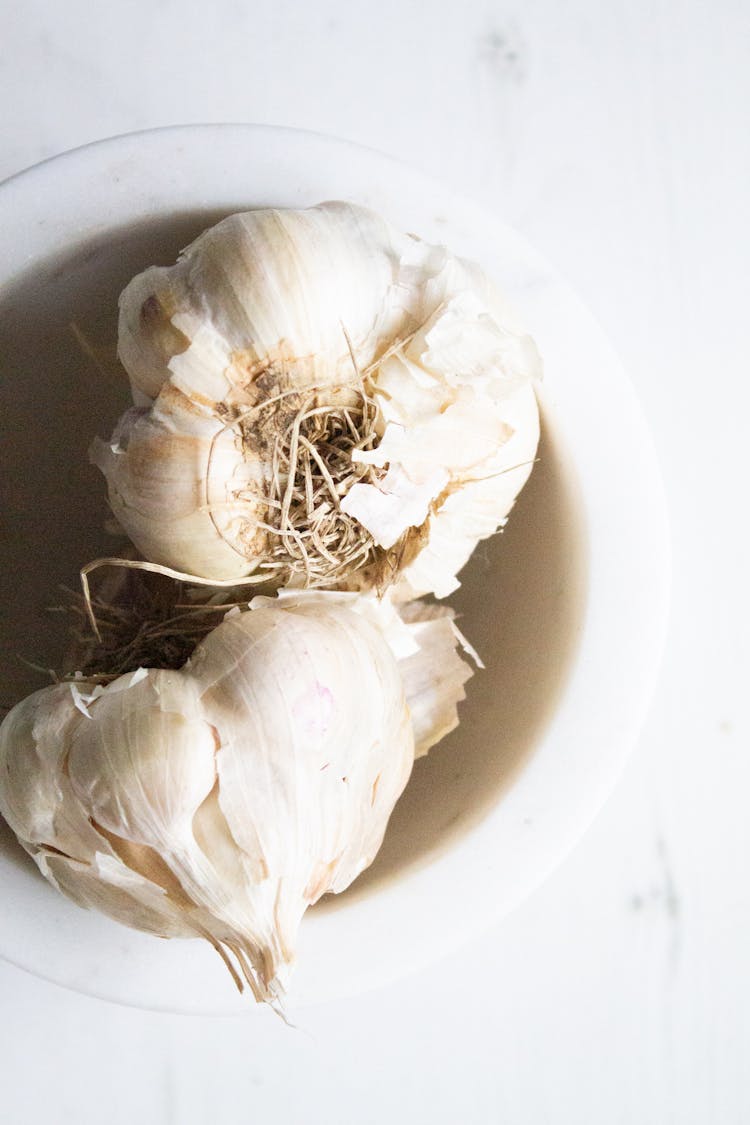This image captures an indoor scene featuring a white marble tabletop illuminated by light from the upper right. Resting on the left side of the tabletop is a white ceramic bowl with a distinct lip around the top edge. Inside this bowl lie two garlic cloves. The cloves exhibit a typical white appearance with some of their outer skin flaking off, revealing dried roots. One clove, more rounded and towards the top, has peeling white skin and visible roots at its center, while the other clove, situated beneath, is more heart-shaped with a pointy end. Shadows cast by the garlic cloves create a contrast against the dark interior of the bowl, emphasizing their texture and form. The overall composition is viewed from above, highlighting the white marble surface and the detailed textures of the garlic.